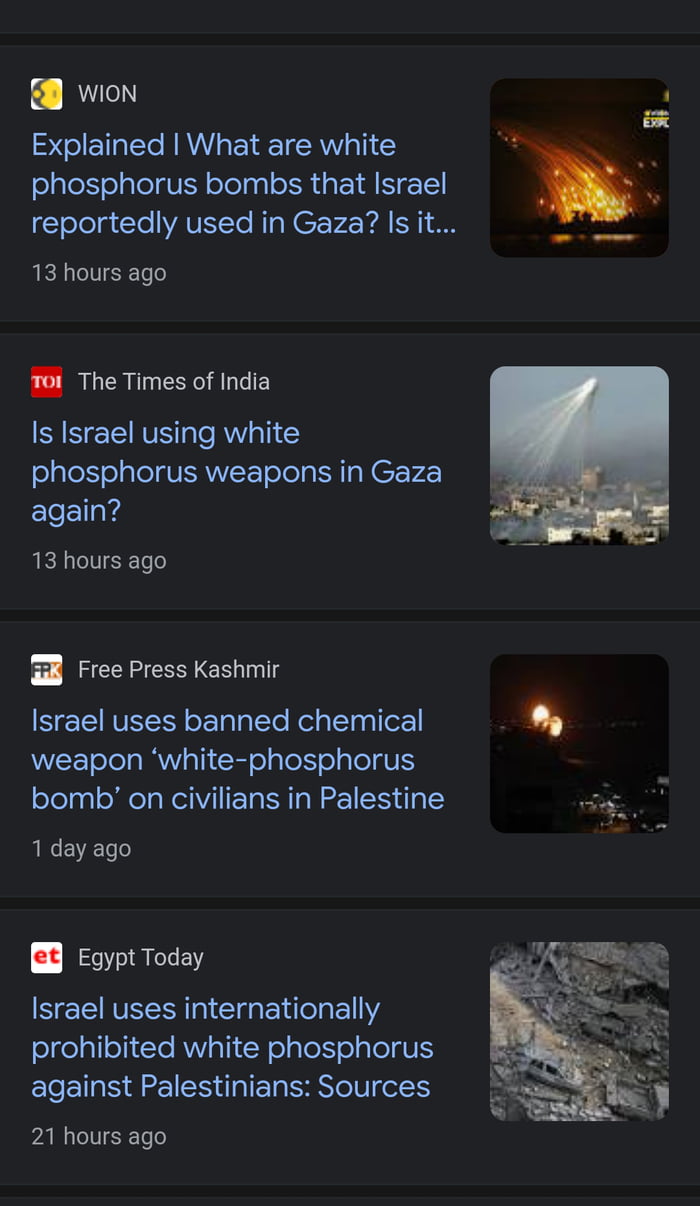This image, captured on a smartphone screen, showcases four distinct news articles covering the controversial use of white phosphorus bombs alleged to have been deployed by Israel in Gaza. Each article is accompanied by a representative thumbnail image. 

At the top of the screen, an article from Yon is titled, "Explained: What Are White Phosphorous Bombs That Israel Reportedly Used in Gaza?" This piece, posted 13 hours ago, features an image with orange and yellow streaks resembling fiery beams.

Below it, The Times of India's article, "Is Israel Using White Phosphorous Weapons in Gaza Again?" also uploaded 13 hours ago, depicts white streams trailing through the sky over a cityscape.

Next, Free Press Kashmir presents "Israel Uses Banned Chemical Weapon, White Phosphorous Bomb on Civilians in Palestine," dated one day ago. The accompanying picture shows bright, fiery objects illuminating the dark sky.

Finally, Egypt Today's piece titled "Israel Uses Internationally Prohibited White Phosphorous Against Palestinians" mentions "sources" and is timestamped 21 hours ago. Its image similarly captures the luminous, incendiary effects in the night sky.

Each article explores the reported use of this banned chemical weapon, reflecting various international perspectives and timeframes.